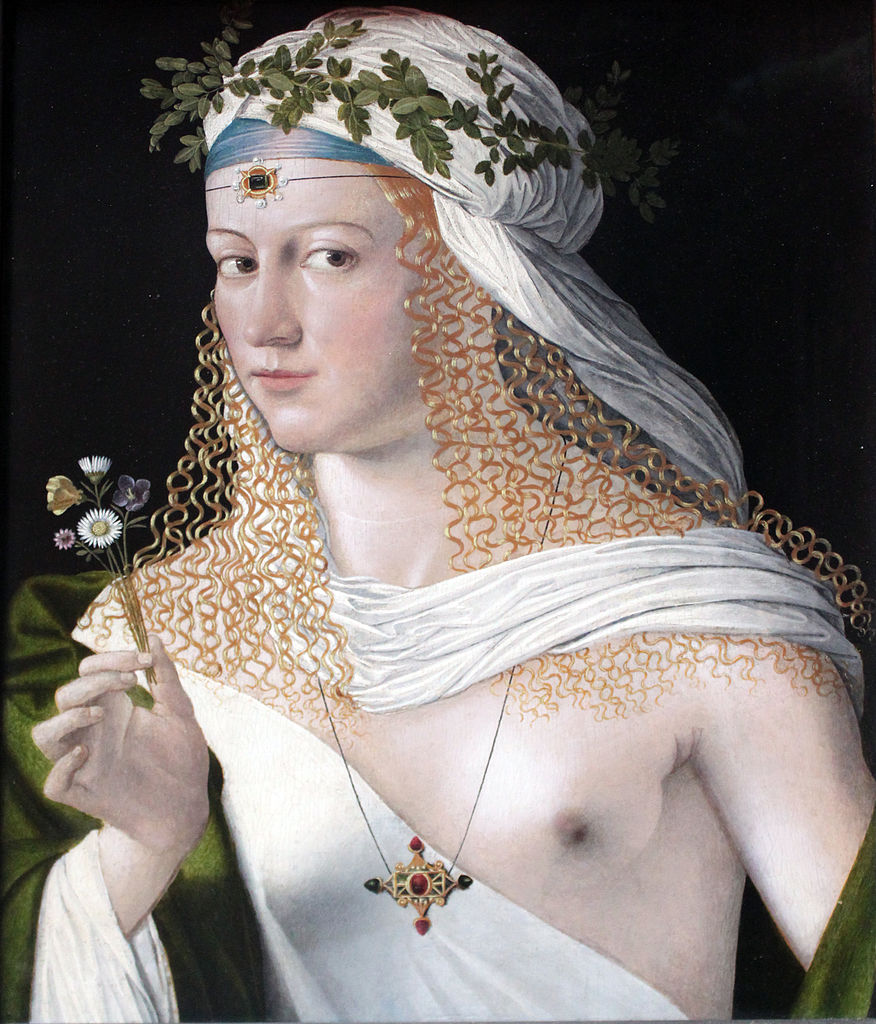This detailed painting, possibly of Renaissance origin, portrays a young individual with a somewhat androgynous appearance, featuring long, meticulously rendered golden curls, possibly with a slight red tint, cascading in fine ringlets from the top of their forehead. The subject is adorned with a delicate headpiece consisting of a white turban or cloth with an interwoven green laurel crown and a distinct blue band just above the forehead.

The attire is a white, semi-transparent tunic draped off one shoulder, leaving the left breast exposed, hinting at masculine features due to its flatness. Draped around the individual’s shoulders is an olive green, silky shawl, adding an elegant touch to the composition. A notable focal point is the ornate jeweled necklace that hangs between their breasts. This necklace features a central oval ruby flanked by teardrop-shaped rubies at the top and bottom, along with black onyx or similar dark gemstones on either side.

Held delicately between the subject's thumb and forefinger is a small bouquet of flowers, consisting of white, purple, pink, and yellow blooms. These flowers, possibly violets and daisies, add to the overall delicate and detailed nature of the portrait. The subject's expression is coy, with a sidelong glance towards the artist, further enhancing the painting’s captivating, graceful essence.